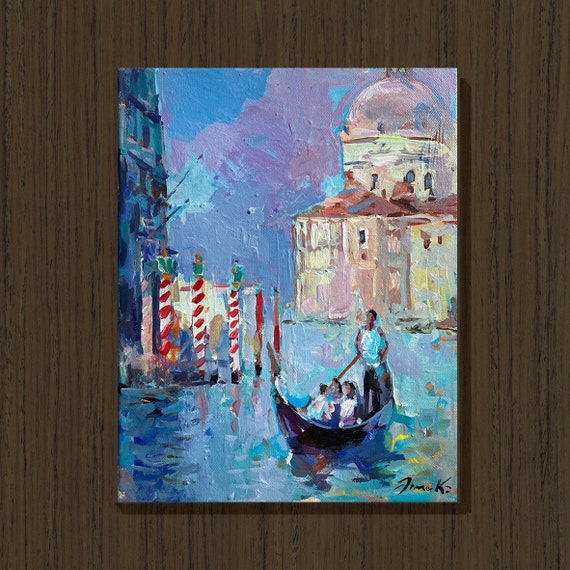This is an image of an acrylic painting hanging on a wall with dark wood paneling. The painting captures a picturesque scene of a Venice waterway, featuring a person rowing a gondola through the canal that winds between the city's buildings. The gondolier, dressed in blue and white, is guiding a couple, possibly parents holding a baby, through the serene water. The hues of the painting are dominated by blues, purples, and whites, creating a hazy, twilight atmosphere suggesting the approaching nightfall.

On the left shoreline, there are holiday-themed decorations, including red and white posts topped with green ornaments, and a deep blue building behind them. Rising into the distance is a mountain, adding depth to the backdrop. Across the waterway, there's another building resembling an observatory with a rounded roof. The painting's style is characterized by broad, wide brush strokes. Jim Kay, the artist, has signed his name in the lower right-hand corner of the canvas.